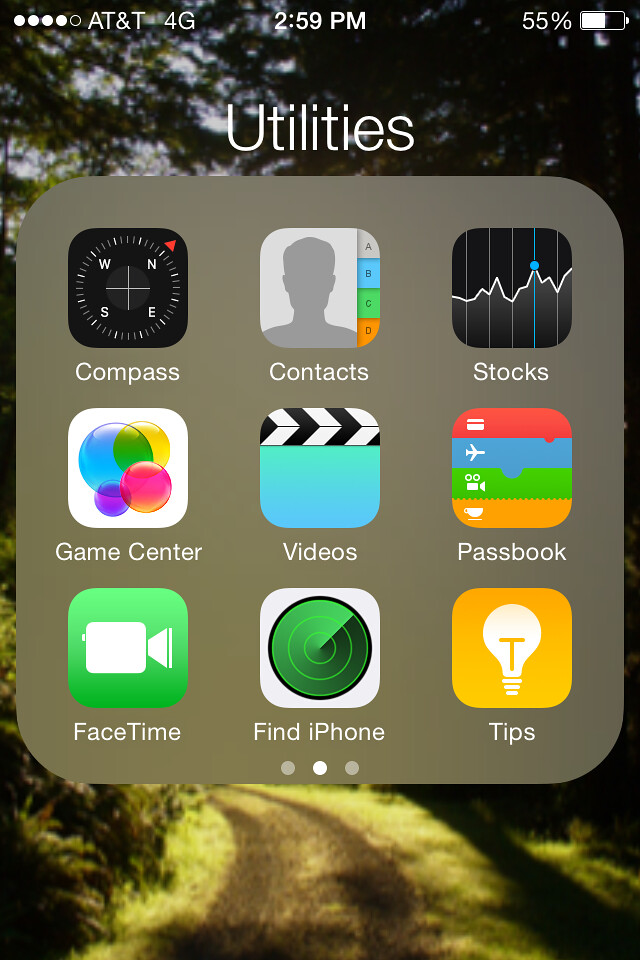The image is a screenshot of a smartphone featuring an AT&T 4G network at the top, with the time displayed as 2:59 p.m. and a battery icon indicating 55% charge. The wallpaper depicts a serene, grassy path winding through a wooded area, resembling an old country road with two faint tire tracks.

The screen is labeled "Utilities" and showcases a variety of icons organized neatly. Starting from the top left, there is a compass widget, followed by Contacts. Next is the Stocks app, represented by a black background with a white bar graph and a blue line. The Game Center icon displays a collection of colorful, transparent bubbles in shades of blue, pink, purple, and yellow, all in varying sizes.

Additionally, there is a Videos icon featuring a classic clapperboard with black and white stripes. The Passbook icon is present, along with FaceTime and Find iPhone widgets. Lastly, there is a Tips widget. This screenshot is from the central page of a three-page home screen setup, as denoted by the pagination indicator at the bottom of the screen.